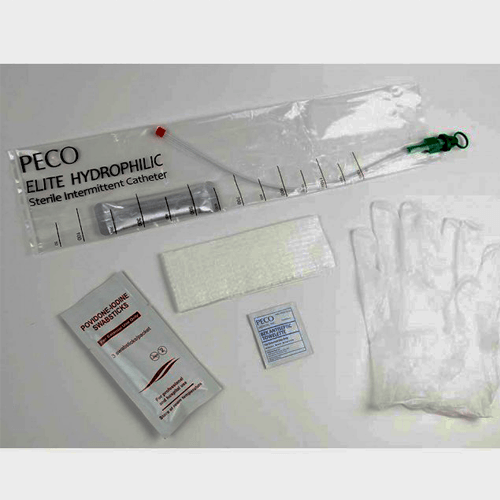The photograph is a horizontally rectangular full-color image dominated by shades of gray. The scene is set against a light gray background on the top and bottom borders, with a gray countertop making up the central background. Featured prominently across the image are five medical items. 

At the bottom right-hand corner, there is a pair of clear, disposable plastic gloves. Adjacent to the gloves on the left, there's a blue packet labeled "PECO," which seems to be a sanitary wipe. Near the center of the image lies what appears to be a piece of gauze or a similar medical item.

Further to the left is another small packet, larger than the blue one, containing iodine swab sticks. Dominating the top part of the image is a long, clear plastic bag with writing on it that reads "PECO Elite Hydrophilic Sterile Intermittent Catheter," clearly showing the catheter enclosed within the bag.